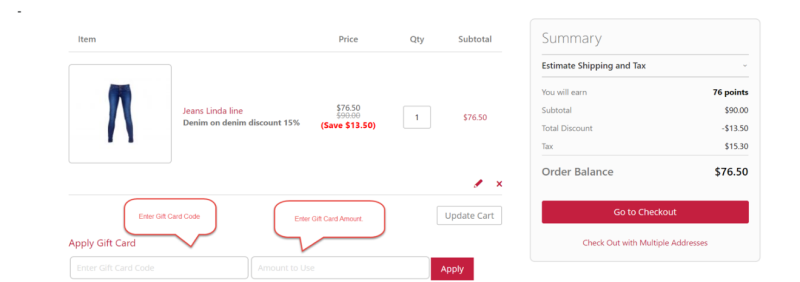This image is a cropped screenshot from an online shopping checkout screen, showcasing a small section of the window. On the left side, there is an itemized list of purchased items, highlighting a singular item: a pair of blue jeans. Accompanied by a small image, the jeans are described as "Jeans Linda Line." The original price of $90 is discounted to $76.50, and in prominent red text, it announces a savings of $13.50. The quantity is set to one, resulting in a subtotal of $76.50. Below the item details, there is an option to enter a gift card number and specify the amount to apply from that gift card, with a red button labeled "Apply."

On the right side, there is a summary of the order. It outlines the points accumulated from the purchase, totaling 76 points. It details the original subtotal of $90, the total discount of $13.50, and the tax amounting to $15.30. Ultimately, the order balance is displayed as $76.50. To proceed with the purchase, there is a prominent red button inviting the shopper to "Go to Checkout."